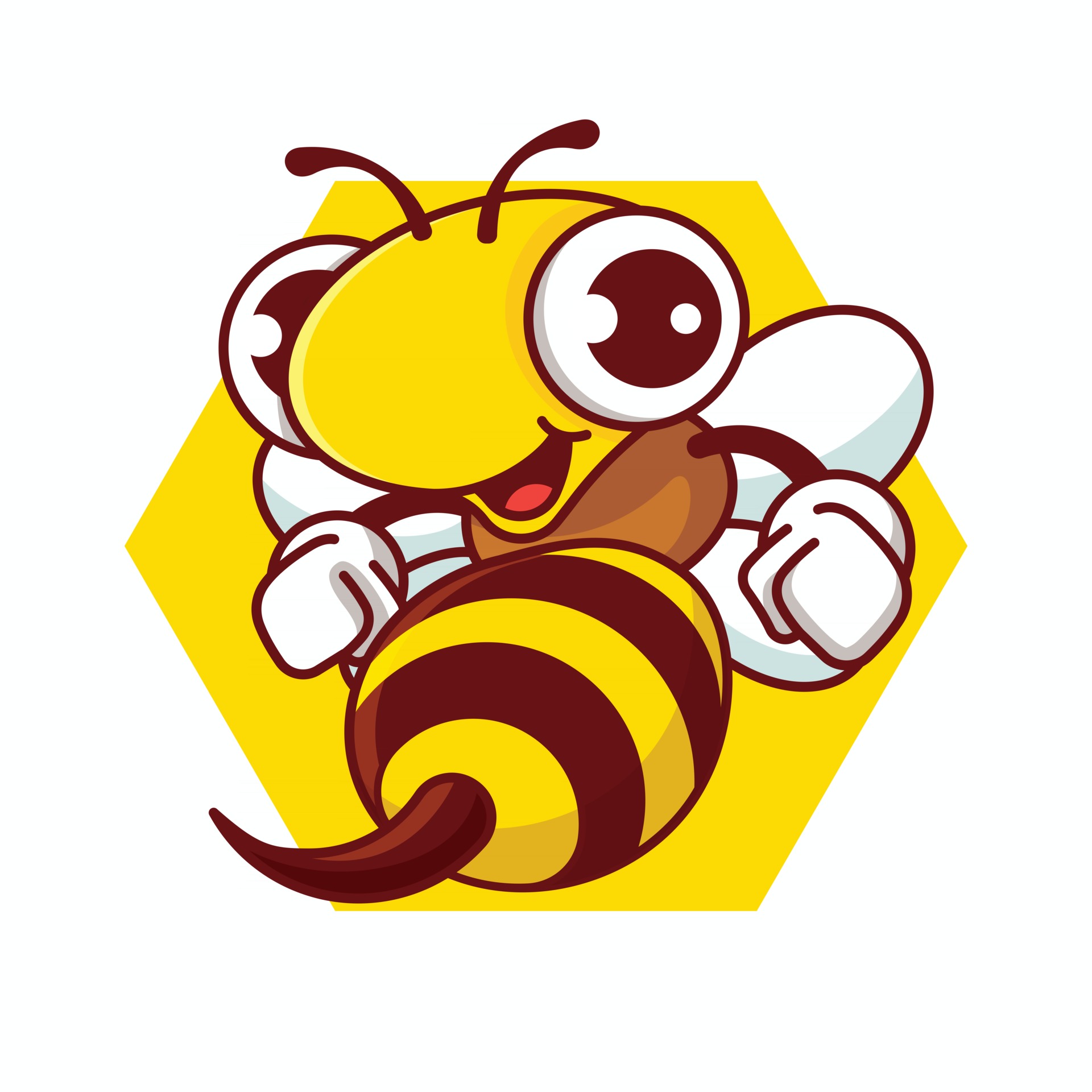This is a detailed graphic illustration of a cartoon bee presented on a bright yellow hexagon background. The bee has an anthropomorphic design, featuring over-accentuated, bulging eyes with brown pupils and a rounded, bean-shaped yellow head adorned with two projecting antennae. The bee has a smiling, happy face with a little red tongue. Its body exhibits the characteristic yellow and brown stripes, transitioning to a predominantly brown abdomen that culminates in a large, prominent stinger angled to the left. The bee appears to be in a three-quarter view, showing its belly and rear end. The arms are simple and tube-like and extend outward, each ending in a fist shape covered by white fingerless gloves, reminiscent of boxing gloves. Four small white wings extend from its back, adding to its animated and cheerful appearance. Overall, the illustration gives an impression of playful exuberance, with no additional lettering or numbers in the background.